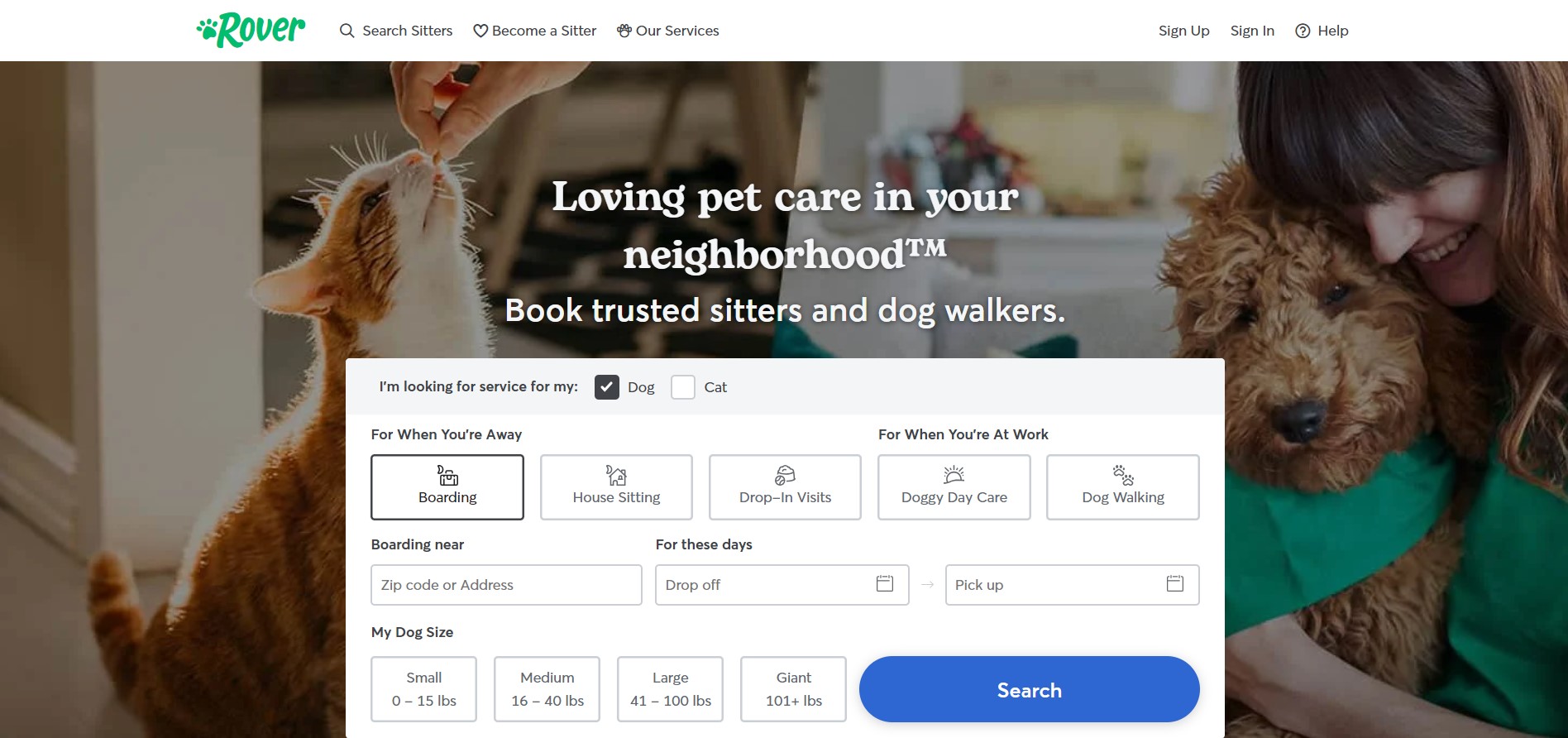The website displayed is Rover, with the name prominently situated at the top of the webpage. The navigation bar includes options labeled "Search," "Search Sitters," a heart icon with the text "Become a Sitter," and a feature called "Air Services" represented by a small tree icon. On the right-hand side of the navigation bar are additional options for "Sign Up," "Sign In," and "Help."

The main image captures a cozy indoor setting, possibly someone's home. On the left side of the image is an orange tabby cat with distinct stripes and white markings on its mouth, nose, and neck. The cat is seated and gazing upwards, focused intently on a hand above its mouth. The hand, which has two fingers extended, appears to be offering the cat a treat or possibly a pill. Alongside this scene, the text reads: "Loving pet care in your neighborhood. Book trusted sitters and dog walkers."

On the right side of the page, there is another image featuring a playful Golden Doodle wearing a green bandana. The dog is being affectionately hugged by a smiling girl with light brown hair and bangs. In the background behind her, a cabinet countertop is visible, holding several items.